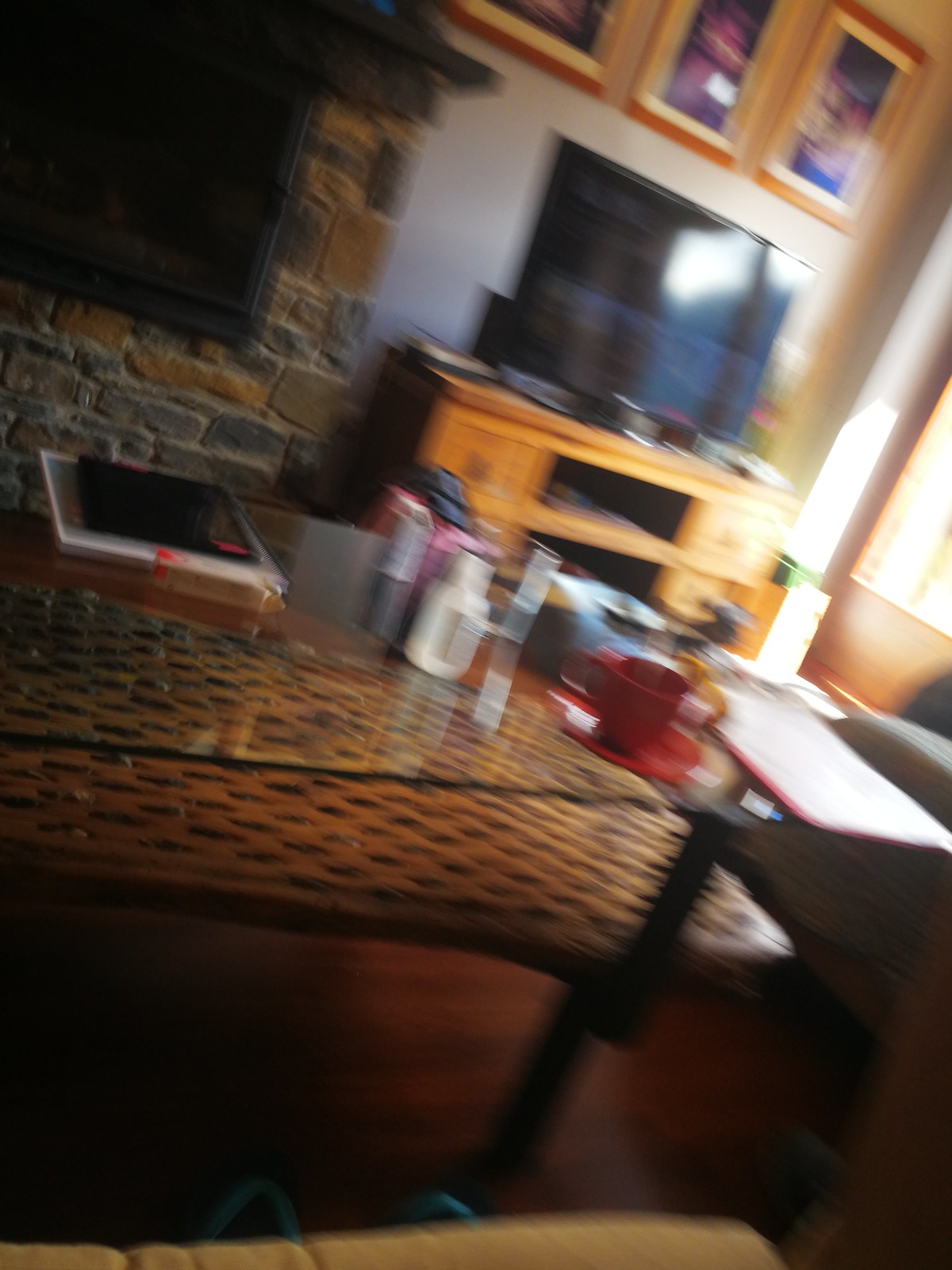This photograph, taken in a family living room, appears slightly blurry, likely because the camera or phone used to capture it wasn't held steady. In the foreground, there's a wicker table with a glass top that holds several items, including notebooks, creams, and a coffee mug. Behind the table, part of a stone fireplace is visible, made of mixed gray and orange stones and partially obscured by shadow. To the right, framed photographs are mounted on the wall, though their contents are indiscernible. Below these, a cabinet with drawers supports a modern television. The corners of two couches can also be seen, indicating a cozy seating area. Natural light filters in from an open window on the right side, illuminating the space with sunlight.